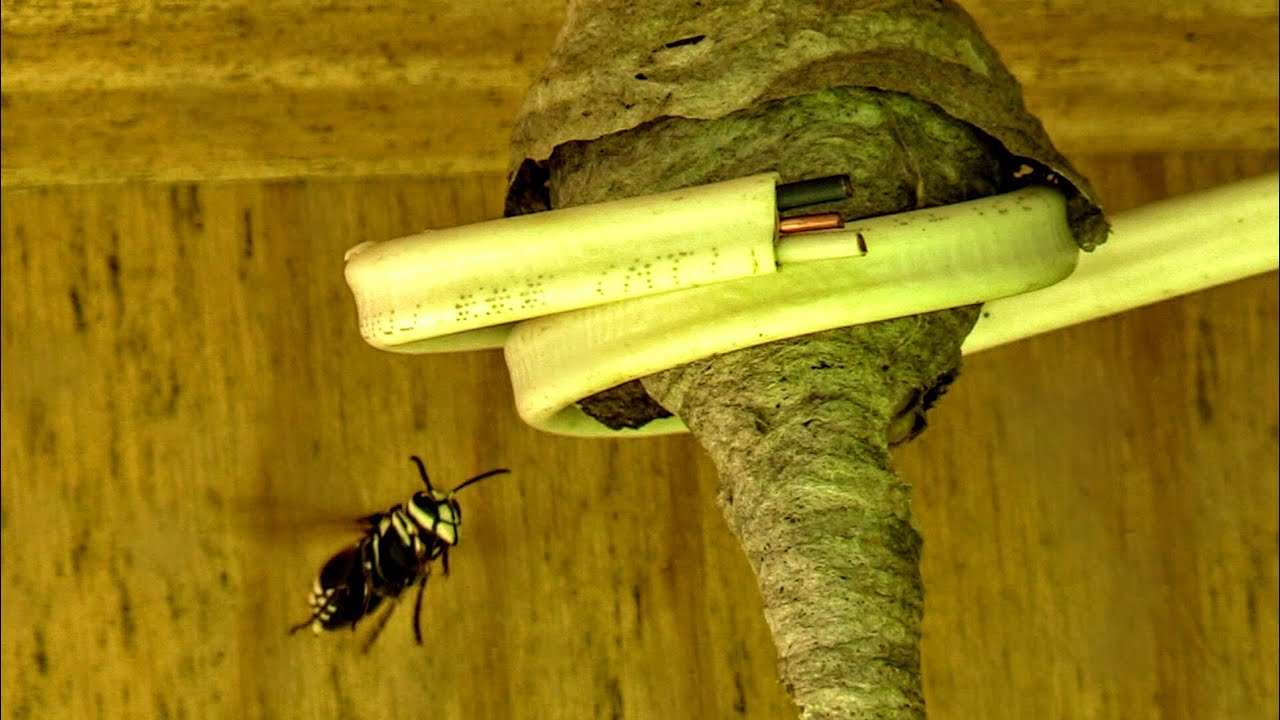This photograph showcases a substantial hornet's nest securely built around a thick, white, plastic-coated cable that encases three distinct wires. The central wire is made of copper, while the wire above it is insulated in black material, and the wire below is wrapped in white insulation. The nest itself is imposing, with a rounded top that tapers into a narrow, conical tail at the bottom. To the left of the nest, a hornet with a striking yellow face, marked with black lines, black eyes, and black antennae, is seen hovering nearby, adding a dynamic element to the scene.